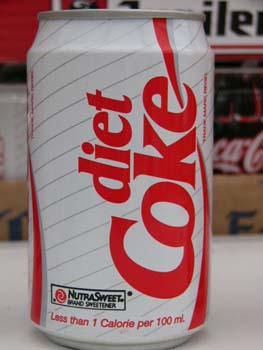This close-up image displays a vintage Diet Coke aluminum can. The can features a predominantly white label adorned with silver stripes running vertically down its length. The Diet Coke logo, written in distinctive red text, is positioned vertically on the can. Near the bottom left of the can, a large black rectangular banner states "NutraSweet brand sweetener," accompanied by an image of a red and white swirled lollipop. Additionally, at the very bottom of the can, in red text, it declares "less than one calorie per 100 milliliters." The can rests upon a white counter. In the background on the right, a portion of the Coca-Cola logo can be seen on a red panel, and above it, there is a white sign with black writing. On the top left of the image, there is a glimpse of what appears to be a red shelf or part of a red sign.